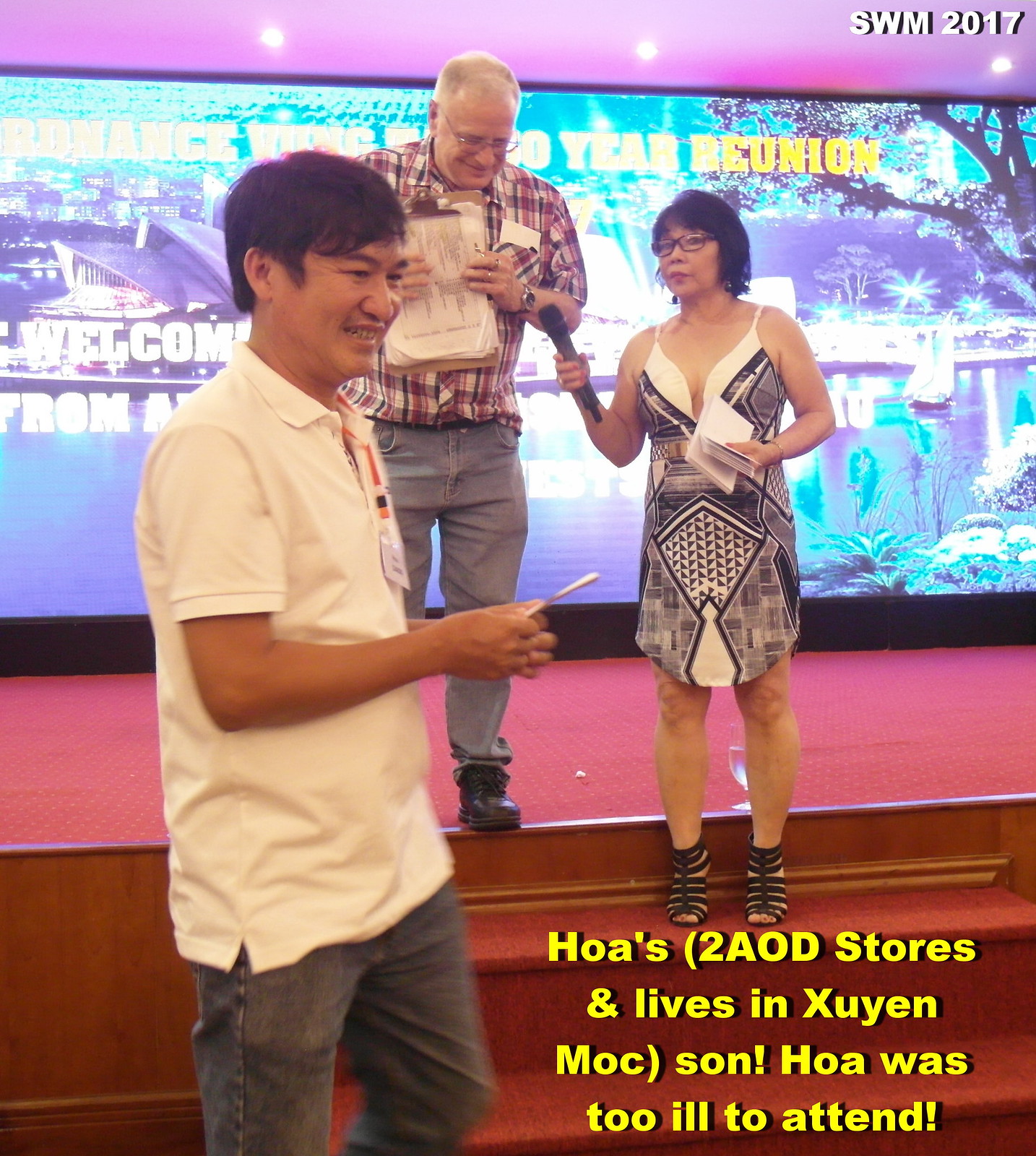In this image, we see three people on a red stage, seemingly at a 20-year reunion event. The backdrop includes an image of a cityscape with a lake, a boat, trees, and buildings. There is partial text behind them that appears to read "HOA's 2AOD Stores and lives in Noizunmak, Son. HOA was too ill to attend," though it is somewhat unclear.

To the left on the stage is a man with short blonde hair, wearing glasses, a red and white short-sleeve plaid shirt, jeans, and black boots. Next to him is a woman holding a microphone. She has short black hair, glasses, and is dressed in a black and white gown with gladiator sandals. In the front, another man is wearing a white polo shirt and gray jeans. The stage and their attire suggest a casual yet respectful atmosphere ideal for a reunion. The visible details and their positions hint at an impending announcement or speech.